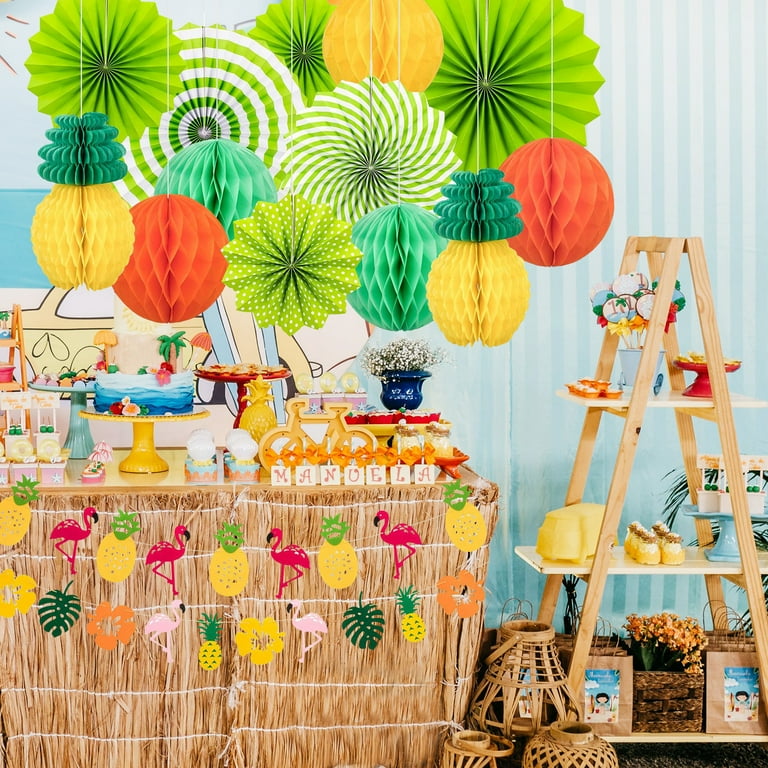The photograph captures a vibrant Hawaiian-themed party scene with a rich array of decorations and intricate details. Set against a light blue and white vertically-striped background, the area is adorned with colorful paper ornaments, including 3D circular balls, pineapples, and spiral pinwheels hanging from strings. Central to the image is a wooden table and a tiki bar draped with grass coverings, accompanied by lively adornments such as pink and fuchsia flamingos, and large palm leaves. The tabletop is laden with cakes, cupcakes, cookies, flowers, and candy, with a V-shaped two-tiered shelf to the side, displaying even more cupcakes and assorted sweets.

To the right of the setup, a ladder decorated with retro-style dishes and pictures serves as an additional display, enhancing the festive atmosphere. The decorations maintain a coordinated palette of greens, yellows, and other bright hues that collectively contribute to the overall cheerful and engaging ambiance. Notably, a yellow pencil drawing of a car subtly appears in the background. Overwhelmingly colorful and detailed, the scene conveys a sense of joyous celebration, underscored by a small sign on the table labeled "Mandel."